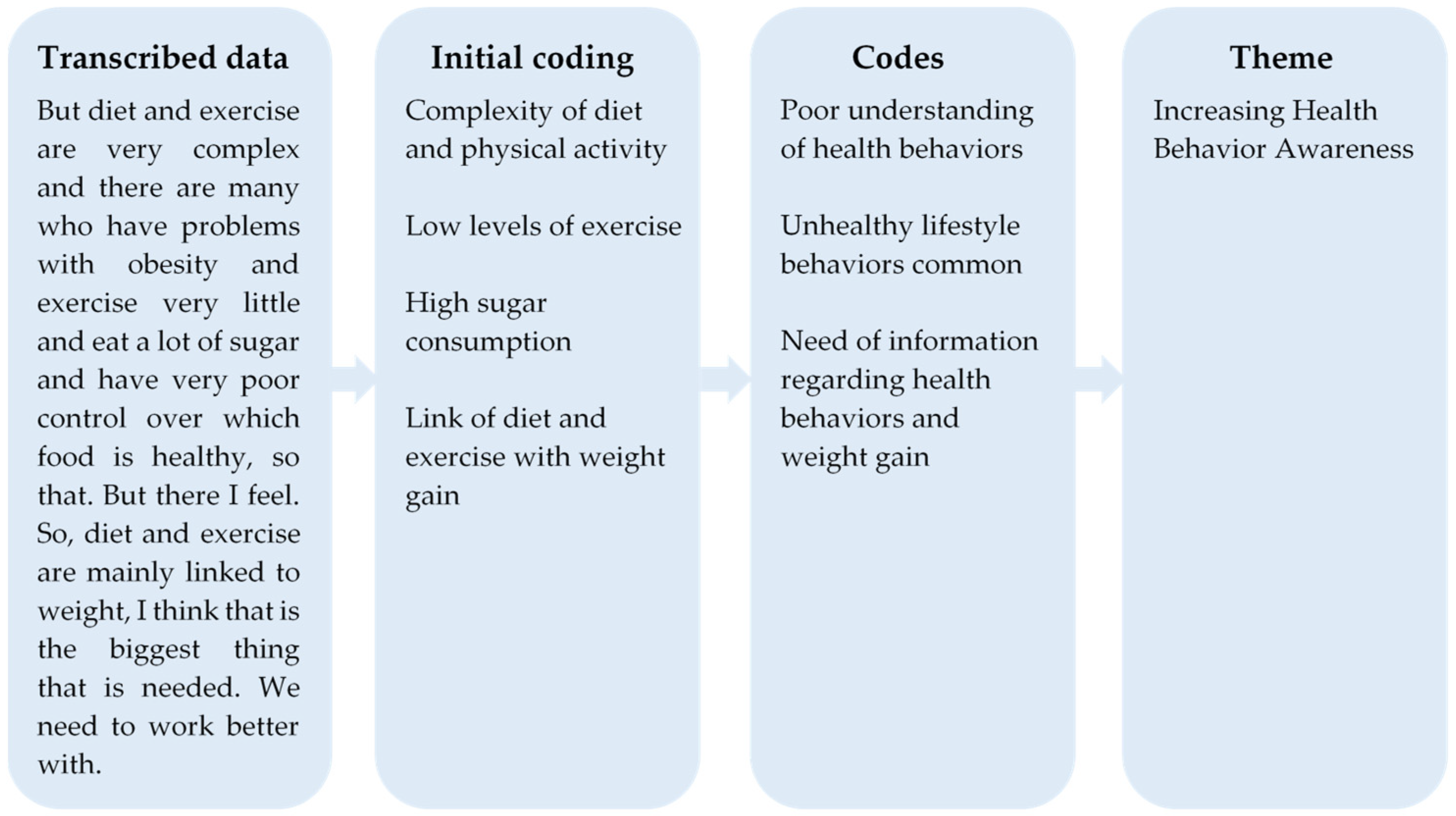This image displays a detailed flowchart set against a white background, consisting of four sequential, long blue rectangular bars with rounded edges, containing text. Each bar leads to the next through blue arrows extending from left to right. 

The first bar, titled "Transcribe Data," highlights the complexity of diet and exercise, noting issues such as obesity, minimal physical activity, high sugar intake, and a poor understanding of healthy foods. The text underneath elaborates on the link between diet, exercise, and weight, indicating the need for improved strategies in these areas.

The second bar, labeled "Initial Coding," lists specific issues such as the complexity of managing diet and physical activity, low exercise levels, high sugar consumption, and the direct connection between diet, exercise, and weight gain.

The third bar, "Codes," identifies broader themes such as a poor understanding of health behaviors, common unhealthy lifestyle choices, and a significant need for better information on health behaviors and weight management.

Finally, the fourth bar, titled "Theme," summarizes the overall goal as "Increasing Health Behavior Awareness," aiming to enhance public understanding and promote healthier lifestyle choices.